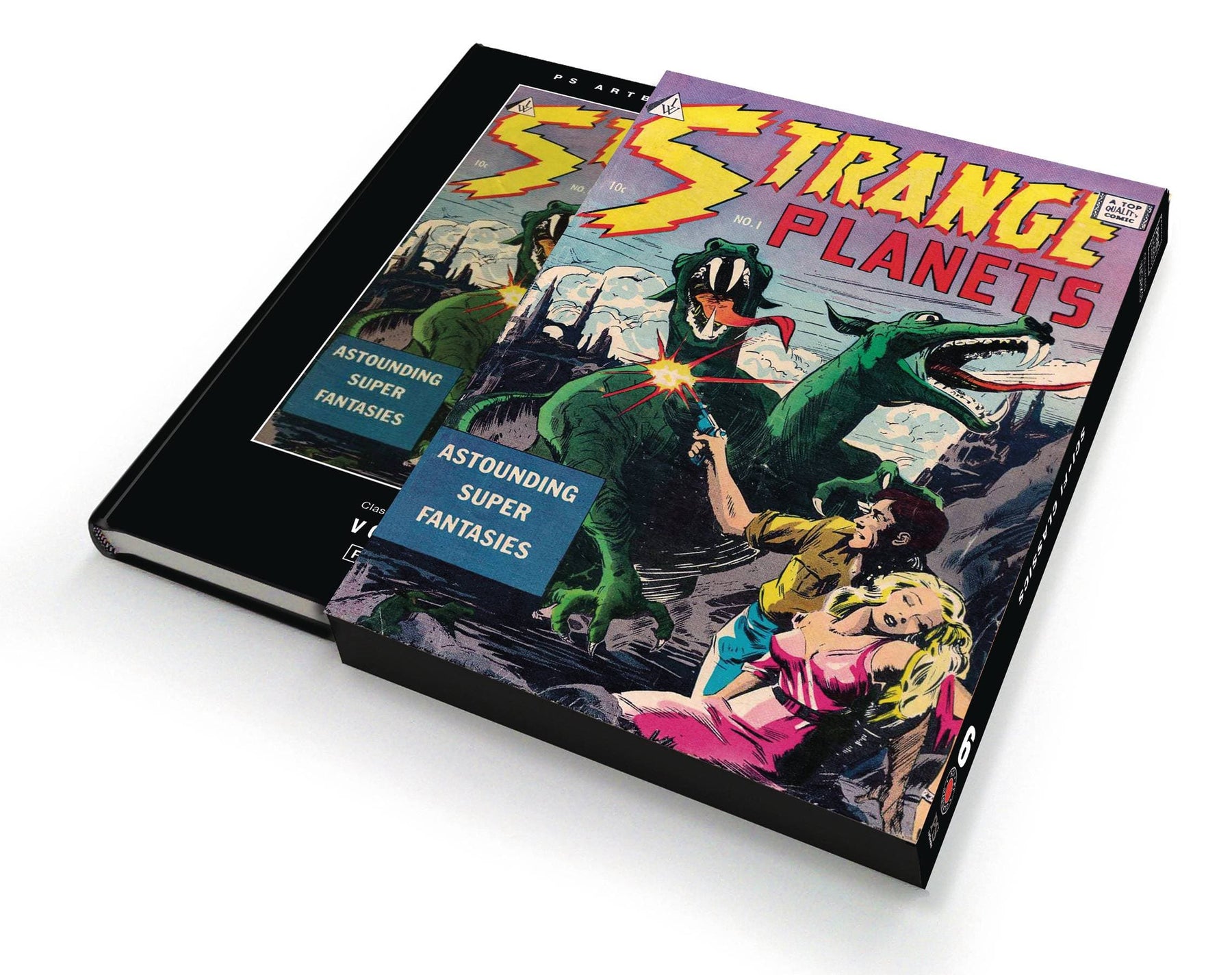The image showcases a vintage comic book, partially encased in a paper slipcover. Prominently titled "Strange Planets" in striking yellow and red letters, the comic also features the subtitle "Astounding Super Fantasies" within a blue box on the bottom left. The dynamic cover art portrays a dramatic scene: a dark-haired man in a yellow shirt and blue pants, aiming a gun at a two-headed dragon lizard beast with ferocious, sharp teeth, as it menaces them from a rocky hill. The man cradles a fainted blonde woman in a pink dress. The slipcover mirrors the vibrant comic book artwork but covers a portion of the underlying hardbound book, which is black with a slightly smaller rendition of the same graphic. The background of the entire scene is stark white, accentuating the intense action and vivid colors of the characters and creatures. Despite tiny, illegible text scattered across the cover, the dramatic visual narrative remains the focal point.